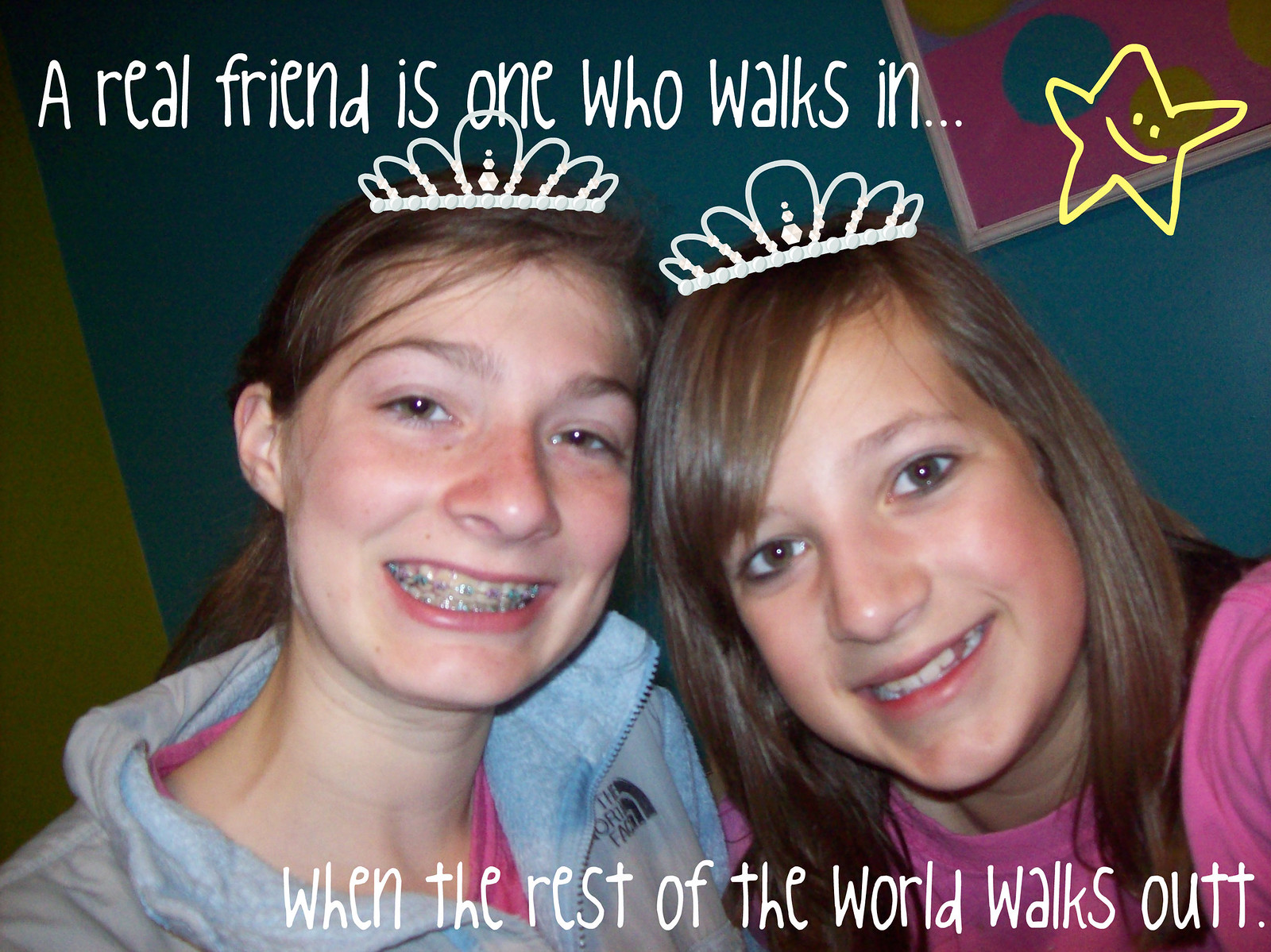This image features two smiling teenage girls with long brown hair and brown eyes, both wearing digitally added princess crowns. The girl on the left has braces and is dressed in a light blue North Face jacket, while the girl on the right wears a pink T-shirt and is missing a tooth. Above their heads is the text, "A real friend is one who walks in," accompanied by a small, hand-drawn yellow star. Below them, the text reads, "when the rest of the world walks out," with "out" notably spelled with two Ts. The background showcases a blue wall, with part of a pink rectangle and bluish square visible in the upper right corner. Both girls are looking directly at the camera, emphasizing their close bond and cheerful demeanor.